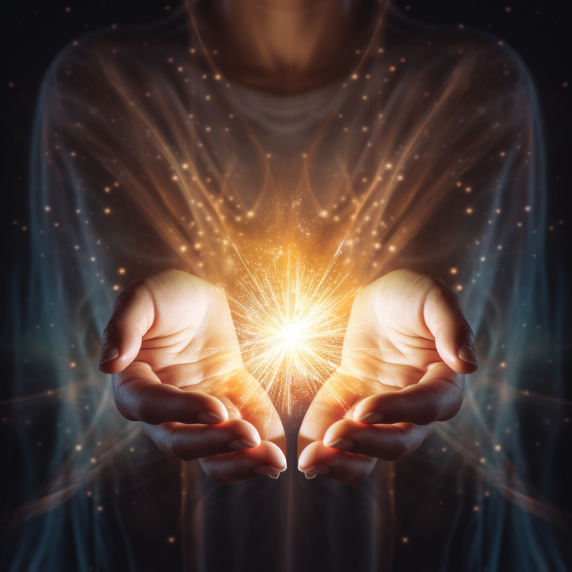In a photorealistic, dark and atmospheric image, a person with their neck and shoulders clad in a diaphanous white gown is partially visible in the background. The focus, however, is on their fair-skinned hands in the foreground, which are extended and cupped as if cradling something precious. Nestled within the hands is a single, bright, star-like light that hovers and emits a radiant glow, illuminating the hands. Surrounding this central light source, myriad smaller, sparkling stars scatter outward, resembling the delicate tufts of a dandelion or intricate spiderwebs of light. This ethereal scene exudes a sense of holding a magical, otherworldly essence, making it reminiscent of a cover for a fantasy or religious book.